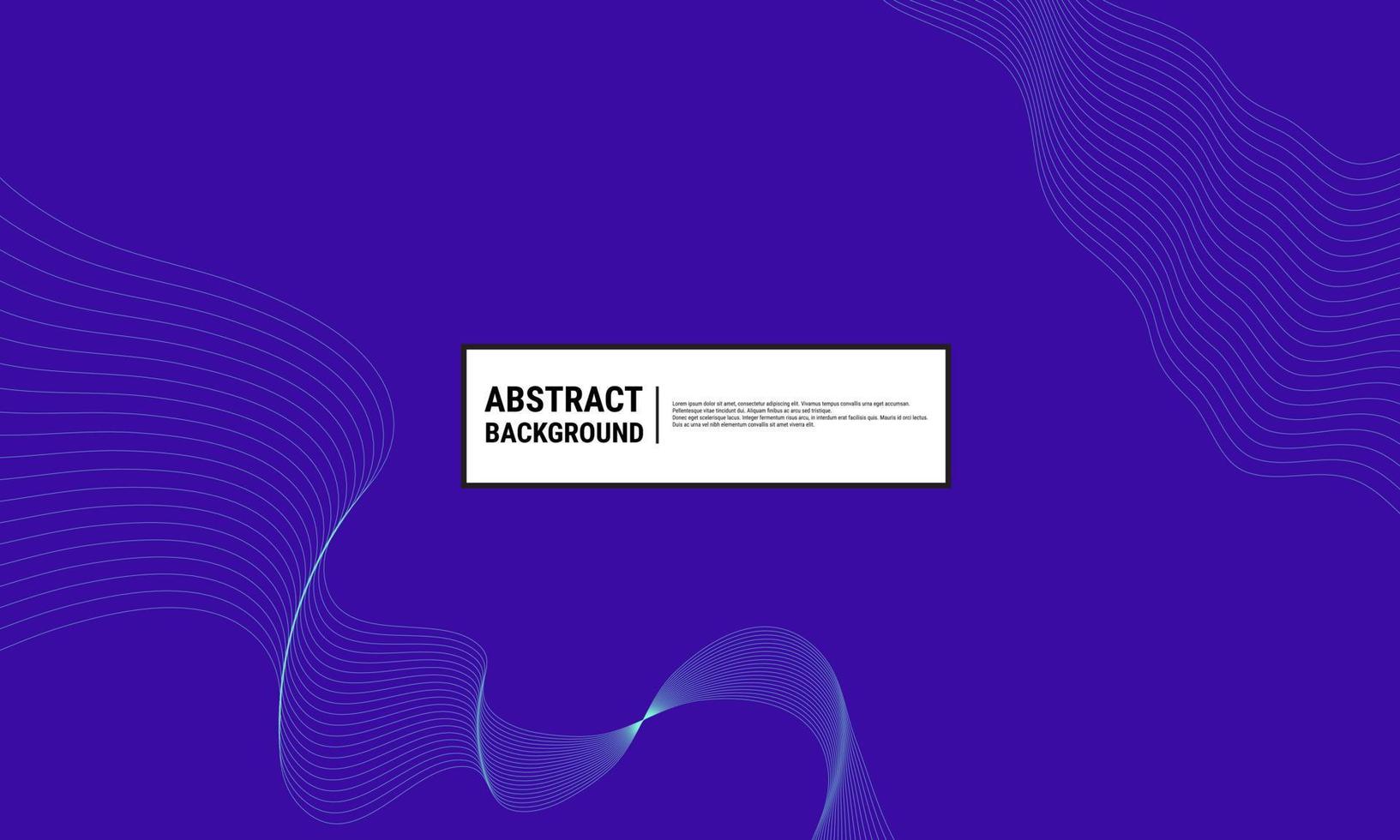The image features a medium purple, slightly wider than tall background with intricate design elements. Wavy, parallel lines in a lighter purple color originate from the lower left and upper right corners, each set approximately 15-20 lines thick, creating ribbon-like, swooping patterns across the background. Centrally positioned is a wide white rectangle, roughly four times wider than its height. Inside the rectangle, in bold black text, the words "Abstract Background" are clearly visible on the left. To the right, there is a paragraph of text rendered in much smaller black font, which is illegible.